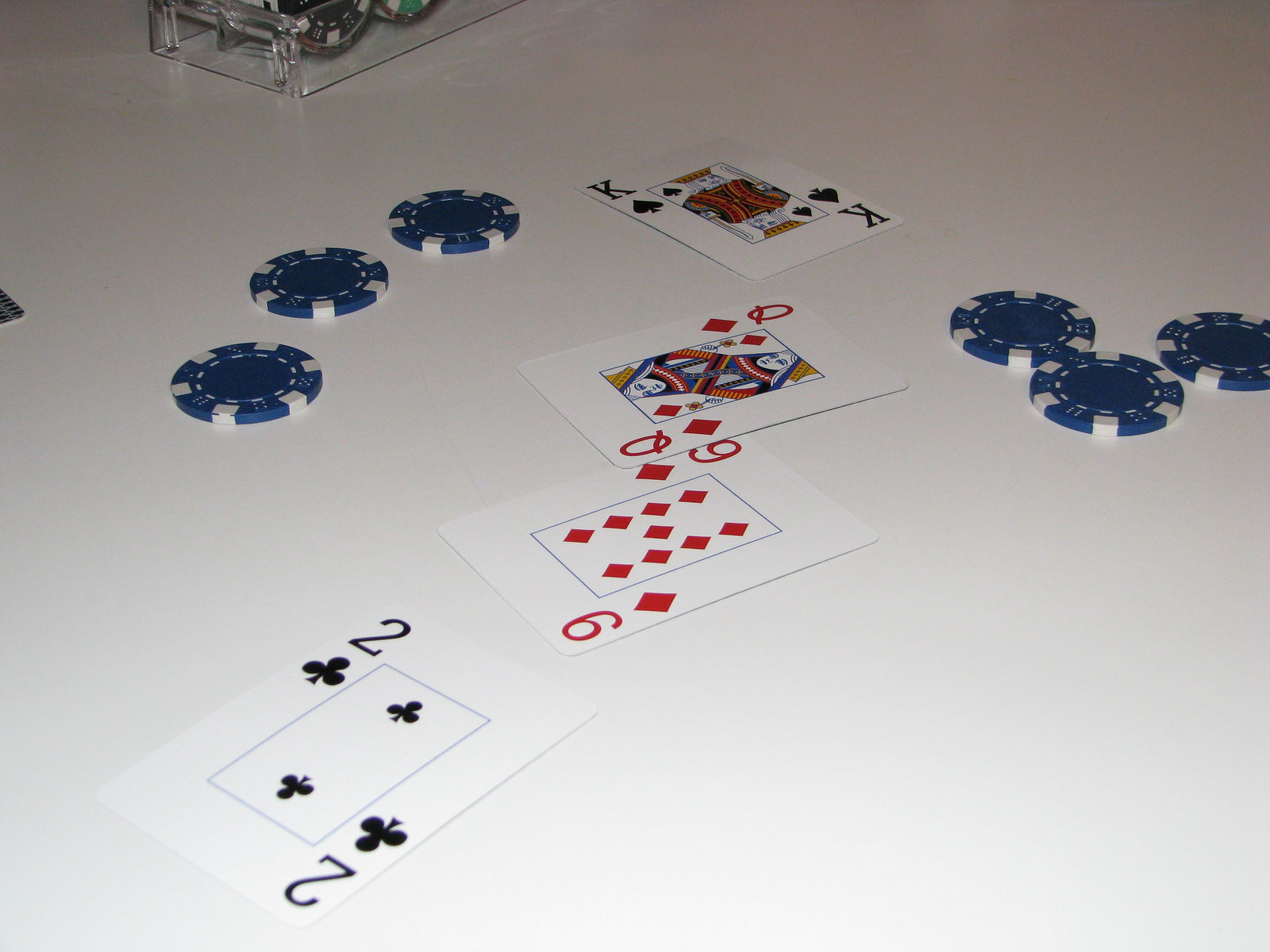The photograph captures an arrangement of four playing cards and six poker chips. The cards, which are turned face up, are the King of Spades, Queen of Diamonds, Nine of Diamonds, and Two of Clubs. In the upper edge of the image, there's a transparent acrylic holder containing additional poker chips. On the left edge, part of another card with a striped pattern is visible. The poker chips present on the table are arranged in two groups of three, featuring a blue center and an alternating pattern of blue-gray and white on the edges. The setting appears to be a broad and large table, likely suggesting a professional or community center environment rather than a typical home game setup. The overall context, indicated by the size of the table and the presence of the poker chip holder, implies a commercial or organized playing venue.